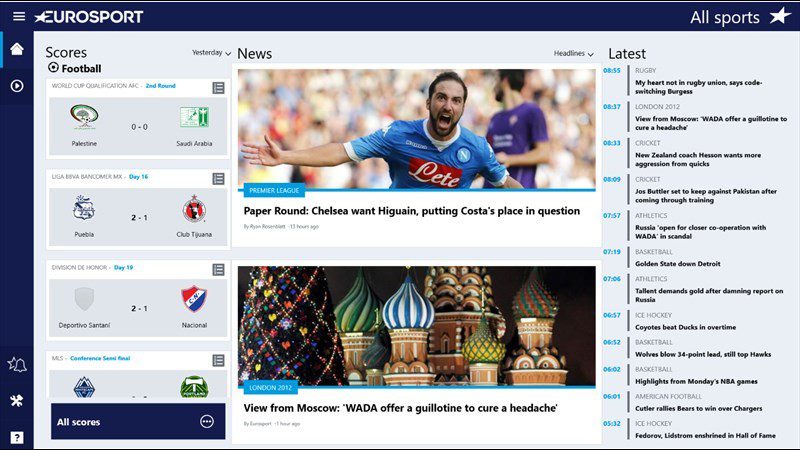The image depicts a webpage from Eurosport, featuring a blue header that prominently displays the Eurosport logo at the top. Beneath the header is a navigation bar labeled "All Sports." The main content is divided into three distinct columns: "Scores," "News," and "Latest."

In the "Scores" section, there are football scores listed, with the match between Palestine and Saudi Arabia being the most legible. The other team names are not clearly readable.

The "News" section features a large image of a soccer player celebrating a goal. The headline below reads, "Paper Round: Chelsea Want Higuain, Putting Costa's Place in Question." Another article below this has a photograph of iconic Moscow buildings, characterized by their mostly brown structures with whimsically colored roofs featuring white, blue, green, and other vibrant hues. To the left of these buildings, a decorated holiday tree is visible. The article is titled, "View From Moscow: WADA Offer a Guillotine to Cure a Headache."

The "Latest" section comprises a list of news titles, each accompanied by a blue timestamp. The first title reads, "My Heart Not in Rugby Unison Says Code Switching Burgess," followed by more vertically aligned headlines. Each title is separated from its timestamp by a thin vertical grey line, maintaining a clear and organized format.